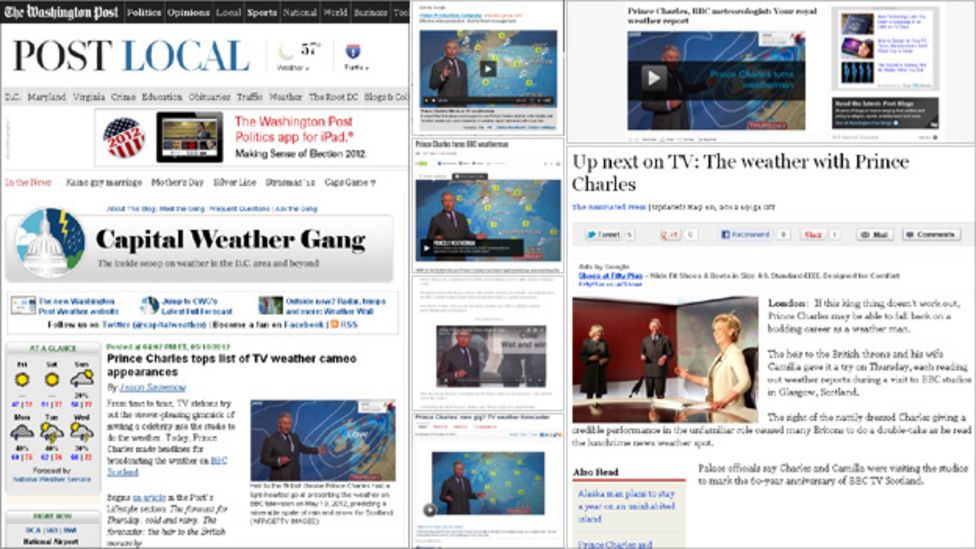The image displays two web pages side by side, both from the Washington Post website. At the top of each page, the Washington Post logo is prominently visible, along with several navigation tabs including "Politics," "Opinions," "Local," "Sports," "National," "World," and an additional tab that is too blurred to decipher. 

Below the main navigation, there is a section labeled "Local" with specific subcategories such as "Maryland," "Virginia," and "Educate." Additionally, there are mentions of "Ambitious Traffic" and other elements, though specific details are unclear.

Prominently dated 2012, one of the pages features a small badge indicating the content is optimized for iPad. Within the content area, there is a focus on political news, as well as a section titled "Capital Weather." Noteworthy is an article spotlighting Prince Charles, listed among top TV weather cameo appearances, with a teaser line reading "Up next on TV, weather with Prince Charles."